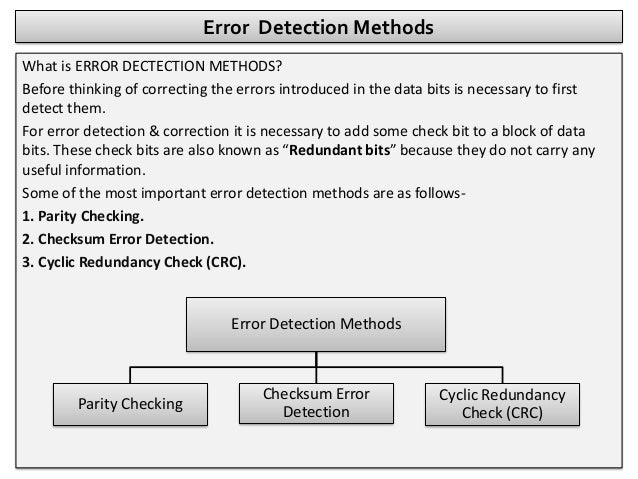The image depicts a gray window, likely a computer screenshot, titled "Error Detection Methods" in black text at the top edge. Below the title, it begins with a heading inquiring, "What is error detection methods?" Despite a typographical error in the heading, the accompanying black text explains the concepts clearly. It states that before correcting errors in data bits, one must first detect them. For effective error detection and correction, additional check bits, also known as redundant bits, are added to data blocks. These check bits do not convey any useful information by themselves but are crucial in identifying errors. The text lists three key error detection methods: Parity Checking, Checksum Error Detection, and Cyclic Redundancy Check (CRC).

At the bottom of the window, a flowchart visually organizes this information. The top rectangular box, labeled "Error Detection Methods," connects via lines to three smaller rectangles positioned below it. These rectangles are labeled "Parity Checking," "Checksum Error Detection," and "Cyclic Redundancy Check (CRC)" from left to right. This structure suggests the hierarchical relation among the various error detection methods.